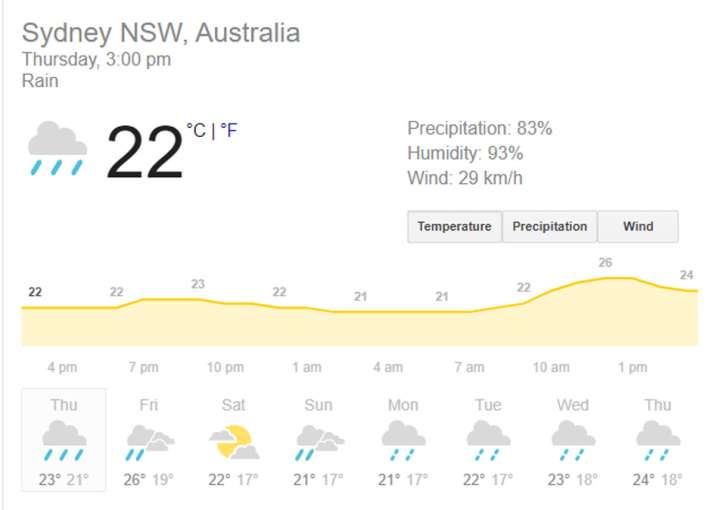The image displays the local weather forecast for Sydney, Australia. As of Thursday at 3 PM, the current weather conditions include rain with a temperature of 22 degrees Celsius. The precipitation level is at 83%, humidity is at a high 93%, and the wind speed is 29 kilometers per hour. 

The day view indicates that the temperature is expected to remain around 22 degrees Celsius until about 1 PM the next day, when it will slightly increase. The weekly forecast shows varying temperatures: 26°C on Friday, followed by 22°C on Saturday, 21°C on Sunday, and 22°C on Monday, with most of these days characterized by rain. The forecast for Saturday suggests cloudy skies with a possibility of dry weather. A toggle is available to switch the temperature display to Fahrenheit.

Additionally, the forecast includes the expected low temperatures, which generally range between 17 and 19 degrees Celsius.